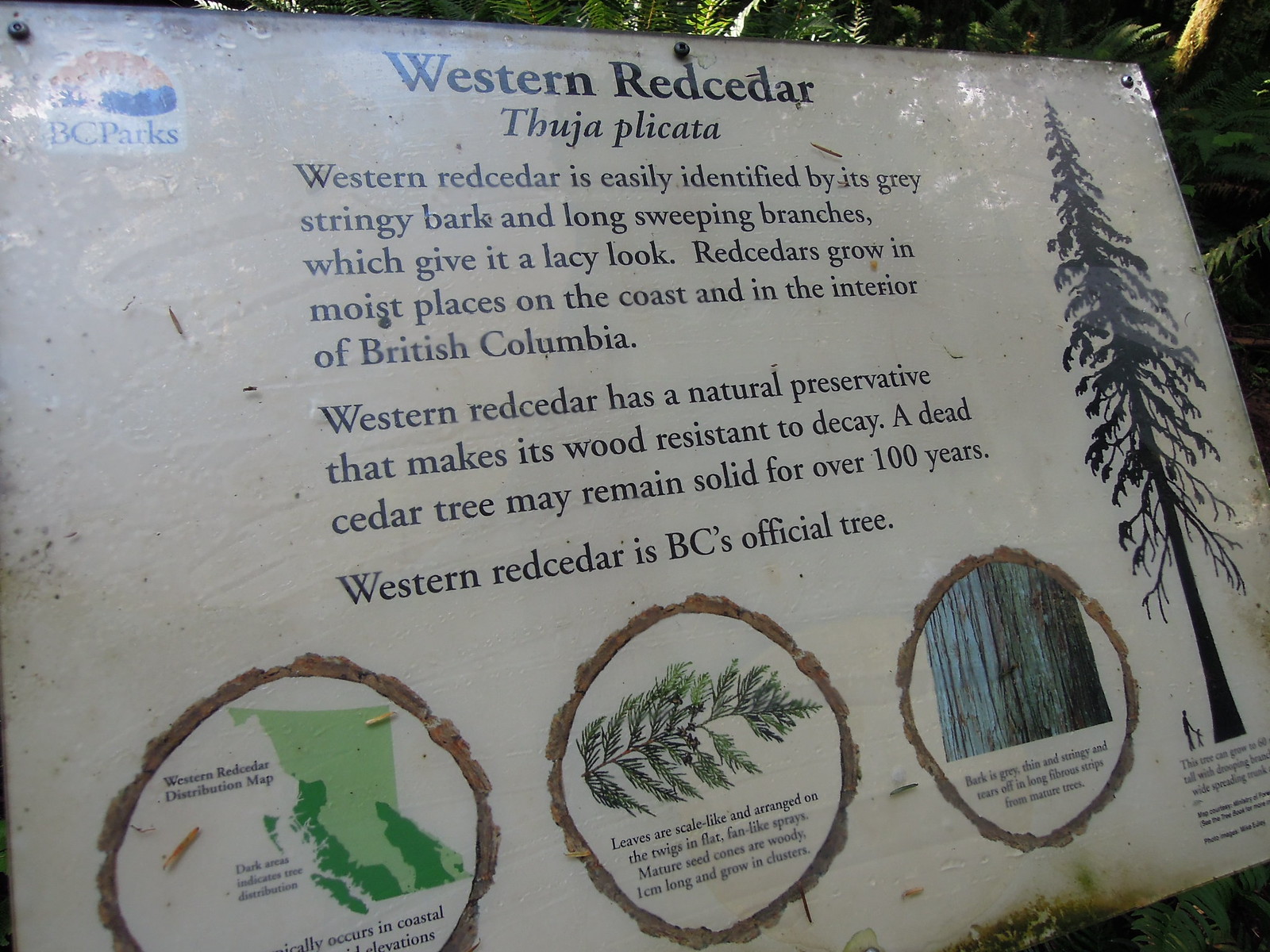In the image, a large, laminated wooden sign stands diagonally, attracting attention with its informative content about the Western Red Cedar (Thuja plicata). Centered in a dense forest setting, the outdoor midday light highlights the vibrant colors of orange, blue, white, black, light blue, light green, and tan, creating a detailed, picturesque scene. The text on the sign describes the Western Red Cedar's key characteristics, including its gray, stringy bark and long, sweeping branches that give it a lacy appearance. The tree thrives in moist areas along the coast and interior of British Columbia, which is its official tree. The sign details the cedar's resilience, noting that its wood is naturally resistant to decay, allowing a dead tree to remain solid for over a hundred years.

Surrounding the main text, the sign includes additional elements: the BC Parks logo in the top right, a map showing the distribution of the Western Red Cedar in British Columbia, close-up images of the tree's leaves, needles, and bark, and a black-and-white illustration comparing the impressive height of the cedar to a man standing at its base, emphasizing its grandeur at about 20 times taller. The detailed and educational nature of the sign enriches the beauty and mystery of the forest surroundings.